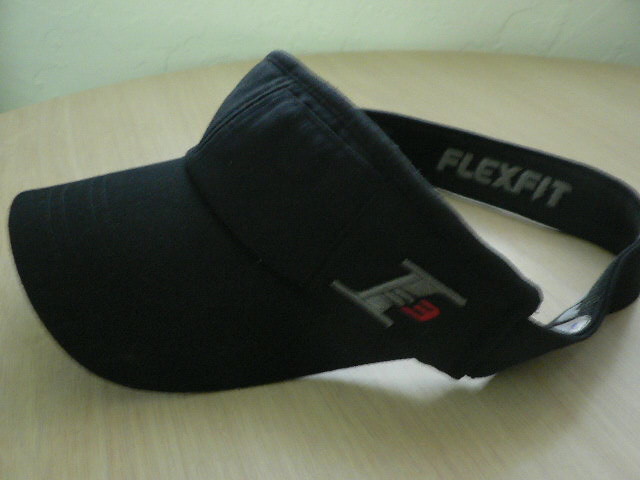The image features a black sun visor cap resting on a light brown laminated tabletop. The tabletop, with its slightly darker brown or greenish lines running through it, provides a neutral backdrop that emphasizes the cap. Positioned against a half-white wall, the sun visor is oriented with its visor pointing to the left. The cap's design includes a prominent strap on the back with the word "FLEXFIT" stitched in gray or white lettering, connecting around to the other side. On the right side of the visor, there is a distinctive red number 3, complemented by a logo featuring two lines at the top and several lines descending down. The sun visor cap lacks a top covering, making it ideal for activities like jogging, where keeping the sun out of one's eyes is necessary.